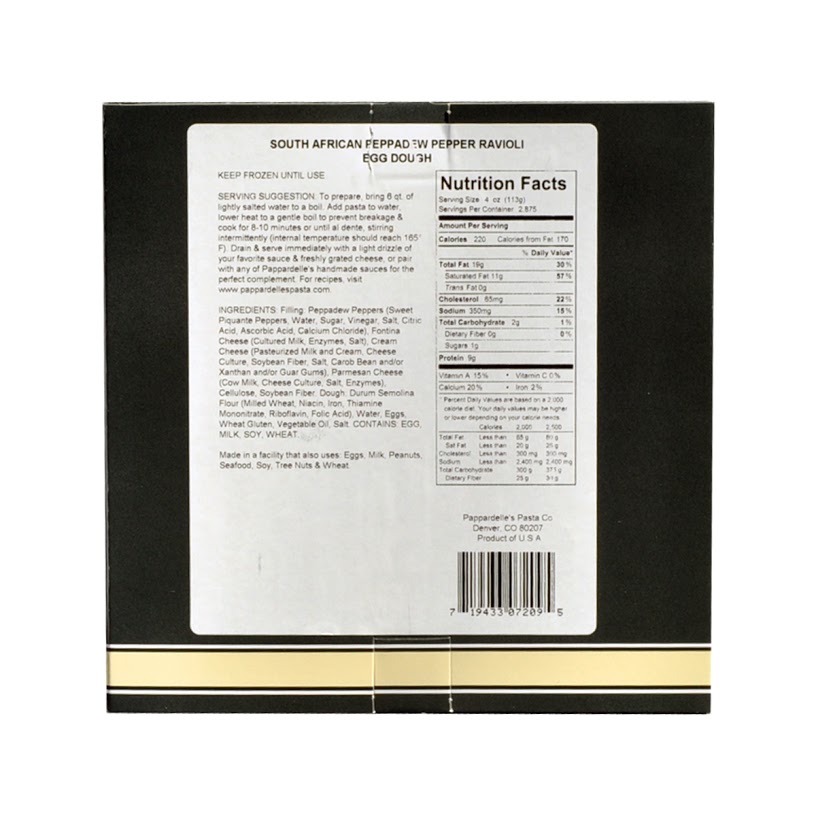Photograph of the back label of a ravioli package. The background is solid black, providing stark contrast to the large, white rectangular label. At the top of the label, prominently displayed in bold black, all-capital letters, is the title: "SOUTH AFRICAN FEED PAD WITH PEPPER RAVIOLI." Beneath this title, the phrase "egg dough" is written in smaller, regular black text. 

On the right side of the photograph, aligned vertically, is a rectangular box outlined in black, labeled "Nutrition Facts" at the top in bold letters. Below this heading, there are two lines of nutritional text, followed by a bold horizontal black line. Additional nutrition information is presented beneath this line, followed by another bold horizontal black line, and even more details below that. Directly under the Nutrition Facts box, a barcode is positioned horizontally.

To the left of the Nutrition Facts box, there are a couple of paragraphs of black text providing additional information about the product. This detailed layout ensures consumers have access to all necessary information about the ravioli contained within the package.